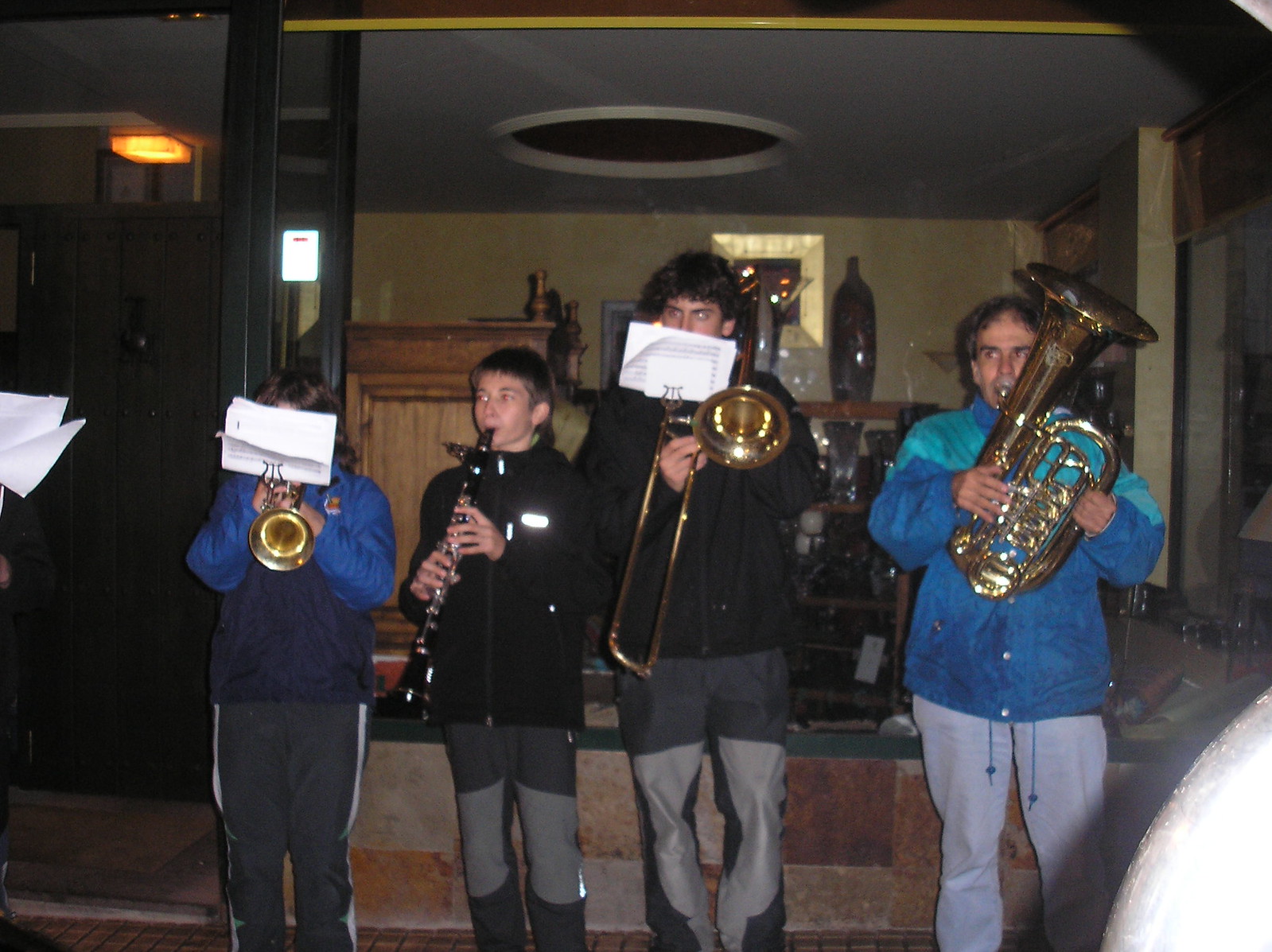The color photograph captures a lively indoor scene featuring four musicians standing in a room adorned with wooden furniture and vases. At the forefront is an elderly man playing a gold tuba-like instrument, dressed in a blue windbreaker jacket and dark pants. To his left are three younger boys of varying ages; the eldest appears to be a teenager holding a trombone, while the middle boy, approximately 10 years old, plays a clarinet. The youngest boy, whose face is obscured by sheet music, plays a trumpet. They are all casually dressed in jackets of blue, navy, and black, paired with pants in various shades of gray and black. The background reveals a large wooden armoire and a noticeable circular feature on the ceiling, adding to the cozy, somewhat cluttered ambiance of the room. Just out of frame to the left, another person appears to be holding music, engaging the musicians' attention.